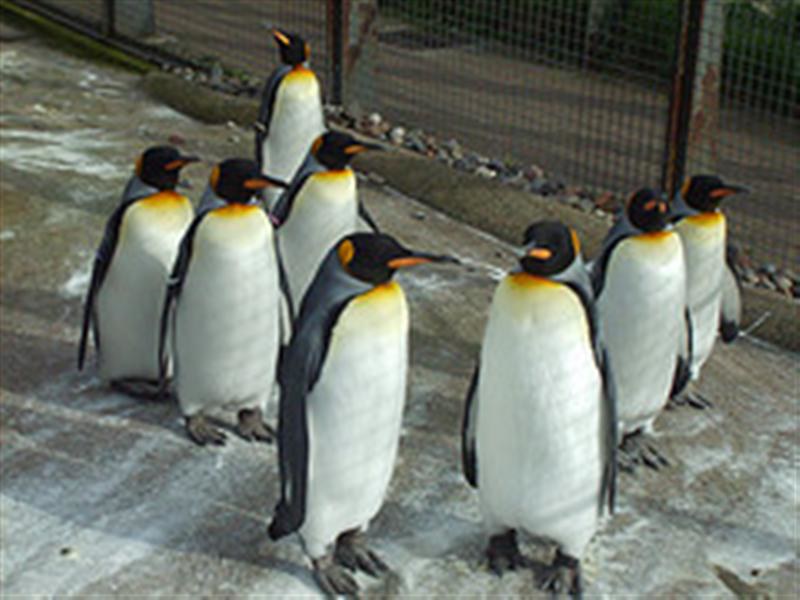This detailed photographic image captures a group of approximately eight emperor penguins standing on a concrete surface within a zoo enclosure. The taupe concrete, streaked with white and lightly dusted with snow and ice, suggests a cold environment. The penguins, who appear nearly identical, boast classic black heads with an orange oval spot at the rear, black upper bills paired with orange lower bills, and glossy black wings and backs. Their eyes are not prominent. Each penguin features a distinctive white chest and belly with a dark yellow splotch at the top of their breasts. They all have black, webbed feet. The penguins are mostly facing different directions, some looking away and one directly at the photographer. The backdrop includes a wire chain-link fence, with rust visible on the metal posts, and some rock placements along the fence. This enclosure setting emphasizes both the containment and the naturalistic elements provided for these majestic creatures.